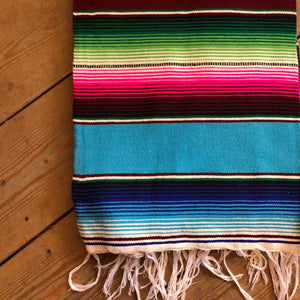This image, which appears as a large thumbnail or a perfectly square photo, depicts a colorful Afghan-style blanket or beach towel laid on a medium brown wood floor with planks arranged at a diagonal angle. The wooden floor features a prominent darker brown grain and black lines marking the separation of each plank. The blanket dominates the view, with intricate horizontal stripes running across it. The pattern starts with black, followed by sequences of dark to light green alternating with white stripes, a horizontal black line, then red to dark red stripes with white in between, a solid medium to light blue section, another black and white stripe, and finally, a mix of dark blue to light blue stripes interspersed with white. The blanket is adorned with beige or white tassels along its lower edge. The vibrant design and detailed patterns on the blanket contrast sharply against the medium wood background, drawing attention to the intricate craftsmanship of the fabric.